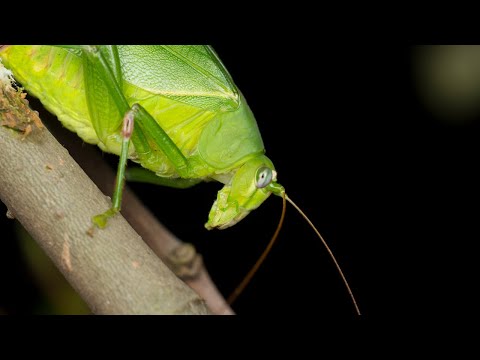This is an extremely detailed, high-quality close-up photo of a vibrant green katydid. The image captures the insect climbing upside down on a tree branch, offering a perfect view of its intricate features. The head, shaped like a football, sports large, prominent eyes and long, thin antennae stretching outwards. The bright green body, resembling the texture and appearance of a healthy leaf, is oval-shaped with slender legs extending from it, and folded wings visible at the sides. You can even make out the delicate details of the katydid’s 'skin' and its small, gripping front foot holding onto the branch. The photo brilliantly showcases the natural beauty and detailed anatomy of this fascinating insect.